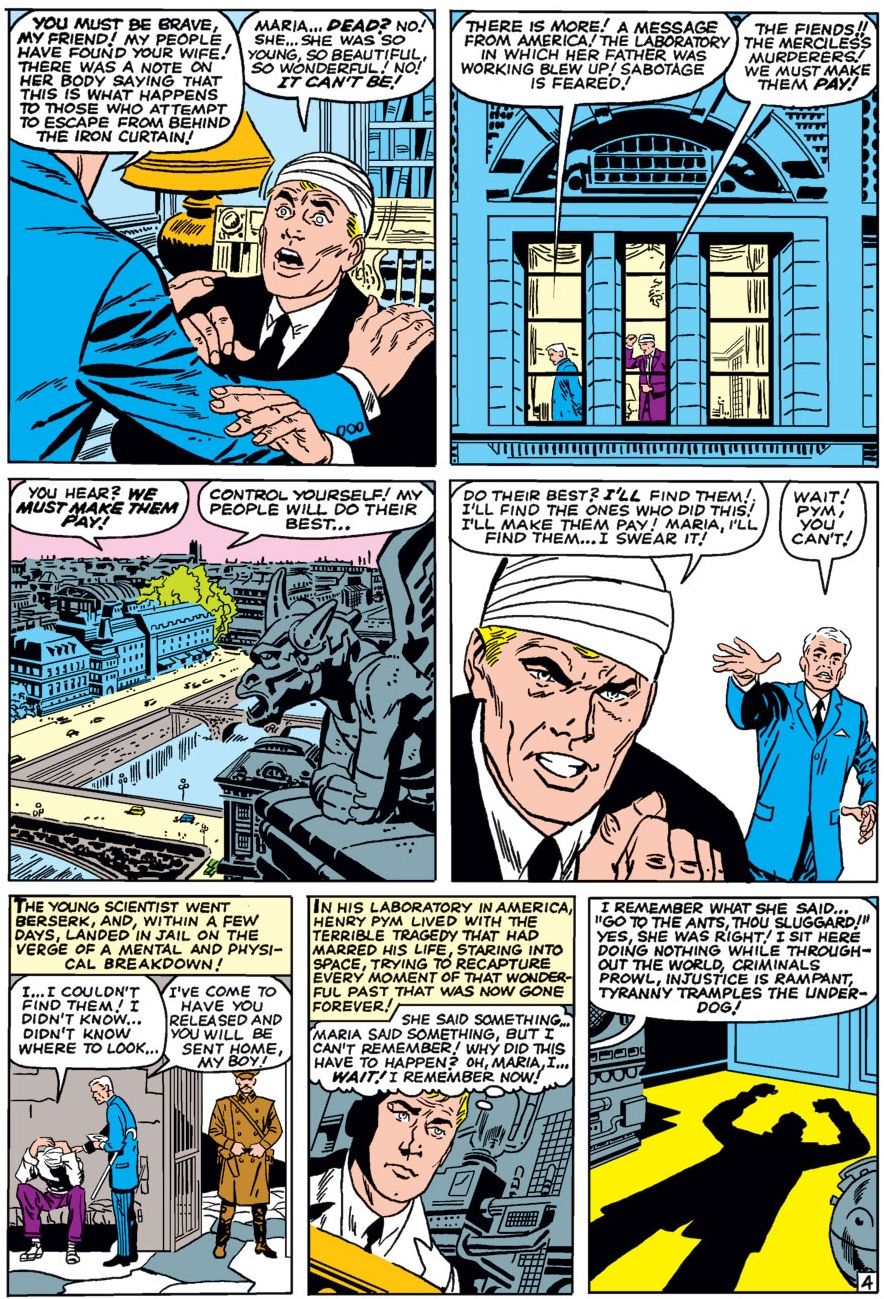This captivating comic book strip page consists of seven distinct panels arranged in three rows: two at the top, two in the middle, and three at the bottom. The color palette prominently features blue, yellow, white, black, with additional accents of purple to differentiate two characters.

**Top Row:**
1. **First Panel:** A dynamic scene unfolds as a man clad in blue pushes back another character dressed in a black suit with a tie and a headband. Two speech bubbles capture their intense exchange.
2. **Second Panel:** Set against the backdrop of a blue building, a man in purple speaks to the man in blue, who wears an identical suit. Both characters communicate through speech bubbles.

**Middle Row:**
3. **Third Panel:** A gargoyle overlooks a sprawling cityscape. Two speech bubbles emanate from the city, suggesting conversations happening off-panel.
4. **Fourth Panel:** The man with the headband, displaying a fierce expression and raised fist, prepares for action. Behind him, the man in the blue suit reaches out, pleading, "Wait, you can't!"

**Bottom Row:**
5. **Fifth Panel:** It appears a man, possibly the one in purple, is being put in jail. The blue-suited man stands beside him, seemingly offering comfort. This panel features three text boxes: two speech bubbles and one narrative box providing context.
6. **Sixth Panel:** A scientist-type character stands within a gray factory, captured in a moment of thought illustrated by a white thought bubble. A narrative yellow text box provides additional scene-setting details.
7. **Seventh Panel:** A shadow cast on the yellow floor hints at a looming figure with a raised fist. Off to the side, a speech bubble references a “dog” or “underdog,” adding an air of mystery to the shadowy scene.

Such rich details and vibrant colors pull readers into the comic's world, making each panel a critical piece of the unfolding story.